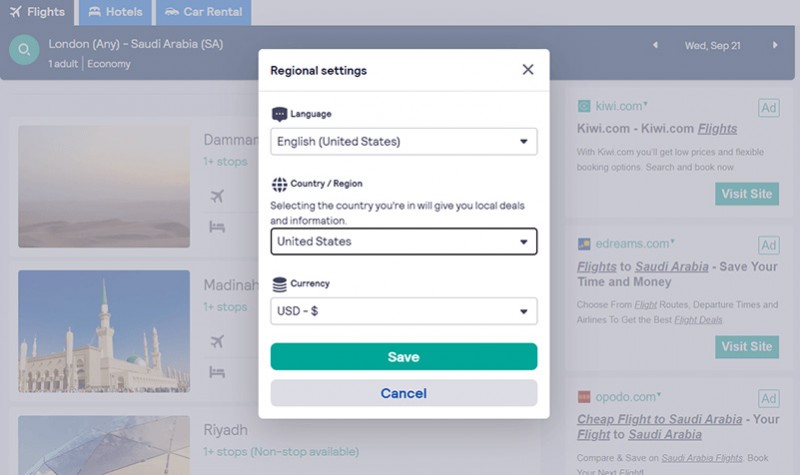The image depicts a detailed screenshot of a travel booking website, focused on booking flights. At the center of the screen, a green circle with a magnifying glass icon highlights the search query "London (NE) – Saudi Arabia (SA)." Below this, it specifies "one adult | economy." 

The top navigation bar includes tabs for "Hotels" and "Car Rental," each with blue icons— a bed for hotels and a car for car rental— while the "Flights" tab shows an airplane icon. On the right-hand side, the date is specified as "Wednesday, September 21st."

A white notification box labeled "Regional Settings" appears at the top-right corner, featuring options for language and regional preferences. It shows "Language: English (United States)" with a dropdown arrow. The "Country/Region" section displays a three-square and six-tile symbol, listing "United States" with another dropdown. The "Currency" section, indicated by a stack of coins icon, displays "USD - $," also with a dropdown. Below these options are green and gray bars for "Save" (in white text) and "Cancel" (in blue text), respectively.

Below the search bar, the first suggested destination is "Dammam," marked in green with "1+ stops." This section includes icons of an airplane and a bed with a gray line beneath. Accompanying the text is a faded image of a desert with a sunset.

Further down, the next suggestion is "Medina," again marked in green with "1+ stops." A similar set of icons and gray line are present, alongside a large building with five spires and a crowd in the foreground.

The final suggested destination is "Riyadh," marked with "1+ stops (nonstop available)" in parentheses. This section features an image of colorful triangular glass structures resembling the exterior of a domed ceiling.

On the right-hand side, three advertisements appear for booking services:

1. **Kiwi.com**: Highlighting low prices and flexible booking options, featuring a "Visit Site" button.
2. **eDreams.com**: Promoting easy flight bookings with a focus on saving time and money, also with a "Visit Site" button.
3. **Opodo.com**: Advertising cheap flights to Saudi Arabia with a call to compare and save, encouraging users to book their first flight with them.

Overall, the interface presents a comprehensive flight booking experience with various destinations and promotional offers tailored to travelers.